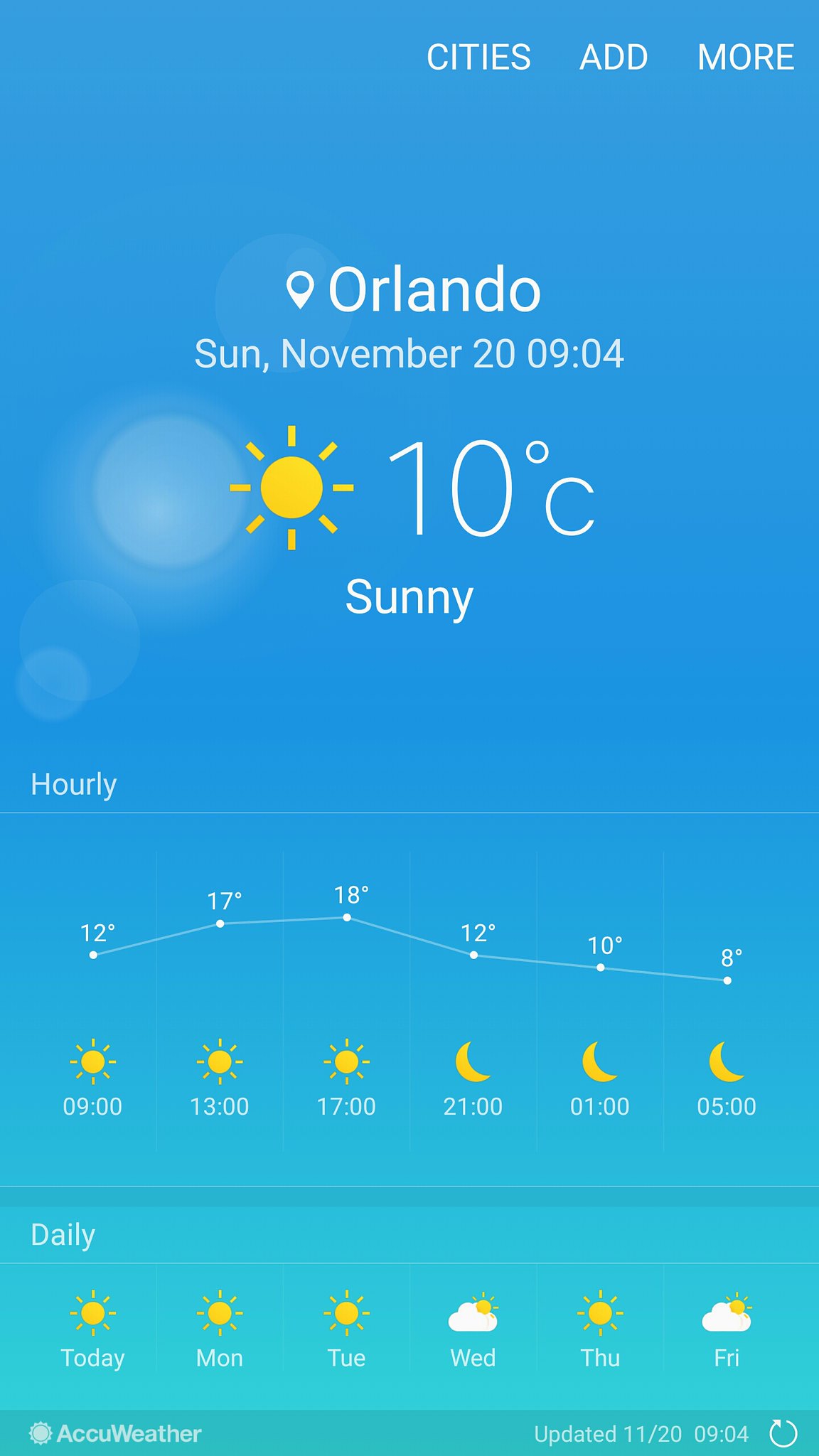This image is a screenshot from a smartphone displaying the AccuWeather app, depicting the weather forecast for Orlando, Florida, on Sunday, November 20th at 9:04 AM. The background of the app is blue, with a sun emoji indicating sunny weather and a temperature of 10 degrees Celsius. At the bottom left of the screen, "AccuWeather" is noted, and the update timestamp "11-20-09:04" is located at the bottom right. Just above these details, a daily weather forecast spanning from Sunday to the following Friday is presented, each day featuring weather icons and respective temperatures in a graph format. The hourly forecast lists times (9, 13, 17, 21, 1, and 5) with corresponding sun and moon icons and temperatures (12, 17, 18, 12, 10, and 8 degrees Celsius). This detailed forecast suggests sunny weather for the upcoming week with mild temperatures for November.